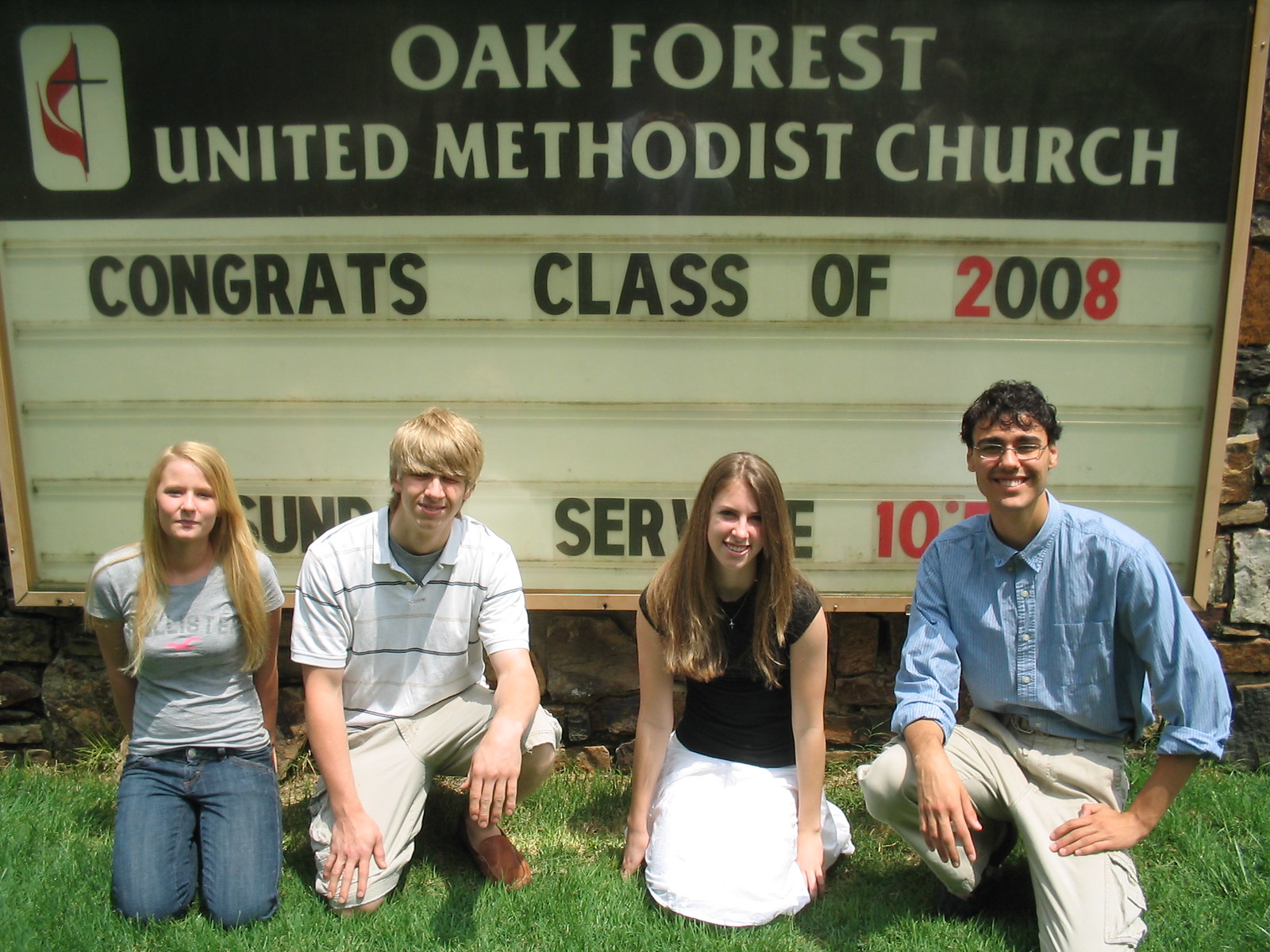In this color photograph taken outside, four young adults are kneeling on green grass in front of a black sign with white lettering that reads, "Oak Forest United Methodist Church. Congrats Class of 2008. Sunday Service 10:30." From left to right, the first person is a young woman with long blonde hair, wearing blue jeans with a black belt, and a short-sleeved gray shirt, both of her hands behind her back. Next to her is a young man with short blonde hair, dressed in gray shorts and a white and blue striped polo shirt with two buttons unbuttoned, kneeling on one knee. To his right, a young woman with long brown hair and a white skirt paired with a black short-sleeved shirt is kneeling on both knees. Finally, a young man with short dark hair, wearing khaki shorts and a light blue long-sleeved button-up shirt with the sleeves rolled up to his elbows, kneels on one knee. All four are looking into the camera and smiling, clearly dressed in their best for this special occasion in front of the Oak Forest United Methodist Church sign.